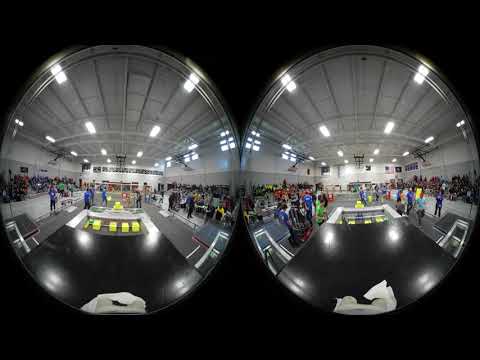This image captures two distorted, round views through clear, lens-like ovals, offering a glimpse into a lively indoor sports event, possibly a ping pong or pickleball game, set inside what appears to be a high school gymnasium. Both views show the same scene but at slightly different times. Visible in the lenses are various details including a central black table surrounded by chairs, fans seated in bleachers to the left and right, and participants dressed in colorful jerseys—some blue, some green—engaged in the game. The gymnasium is well-lit with bright, rectangular fluorescent lights hanging from the ceiling, which is supported by silver bars, and the walls are painted white. Additionally, some individuals are seen capturing the event with cameras. The background beyond the lenses is black, further emphasizing the focal points within the ovals.